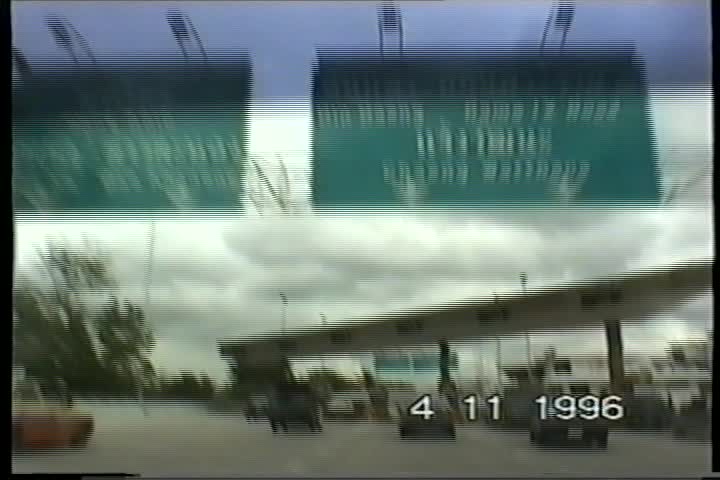The image captures a bustling toll bridge scene under a pristine white overhang. The sky above is dotted with fluffy white clouds, and lush green trees frame the setting, adding a touch of nature to the urban landscape. Dominating the view are large green road signs emblazoned with white writing, offering directions to the drivers below. The multiple lanes are filled with several cars, suggesting a busy moment at the toll. At the bottom of the picture, a timestamp reading "4-11-1996" in white writing situates the image in time. The lanes stretch out ahead, converging under a substantial roof that houses numerous small toll booths. Further along the road, additional large green signs provide guidance for the journey ahead.